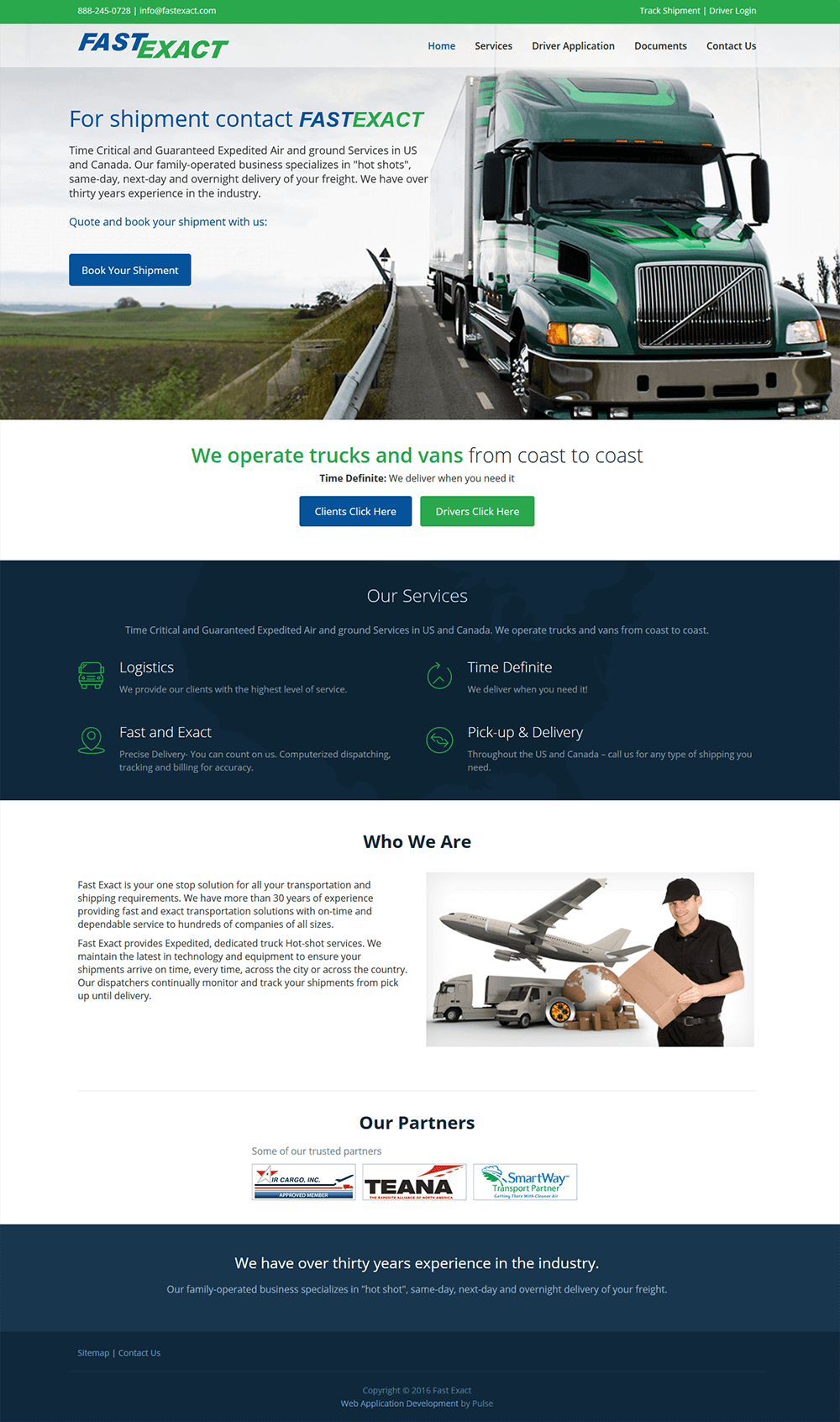This image is a detailed snapshot of the FastExact website, known for its coast-to-coast shipping services. The website features a vibrant green banner at the top, under which several navigational tabs are available for users to explore different sections. Central to the website's body is an impactful image of a large green big rig truck, symbolizing FastExact's extensive transport capabilities. Below this image, a tagline proudly states, "We operate trucks and vans from coast to coast," reinforcing the company's nationwide service range.

Additionally, the website includes a blue button labeled "Cargo, click here," presumably directing users to information or services related to cargo transport. There's also an indistinct green tab whose label is not clearly readable. Below these elements, a blue banner titled "Our Services" provides a comprehensive breakdown of the company's offerings, including logistics, fast and exact time, and pickup and delivery options.

FastExact emerges as a pivotal player in the shipping industry, dedicated to transporting various products across the nation with precision and reliability.